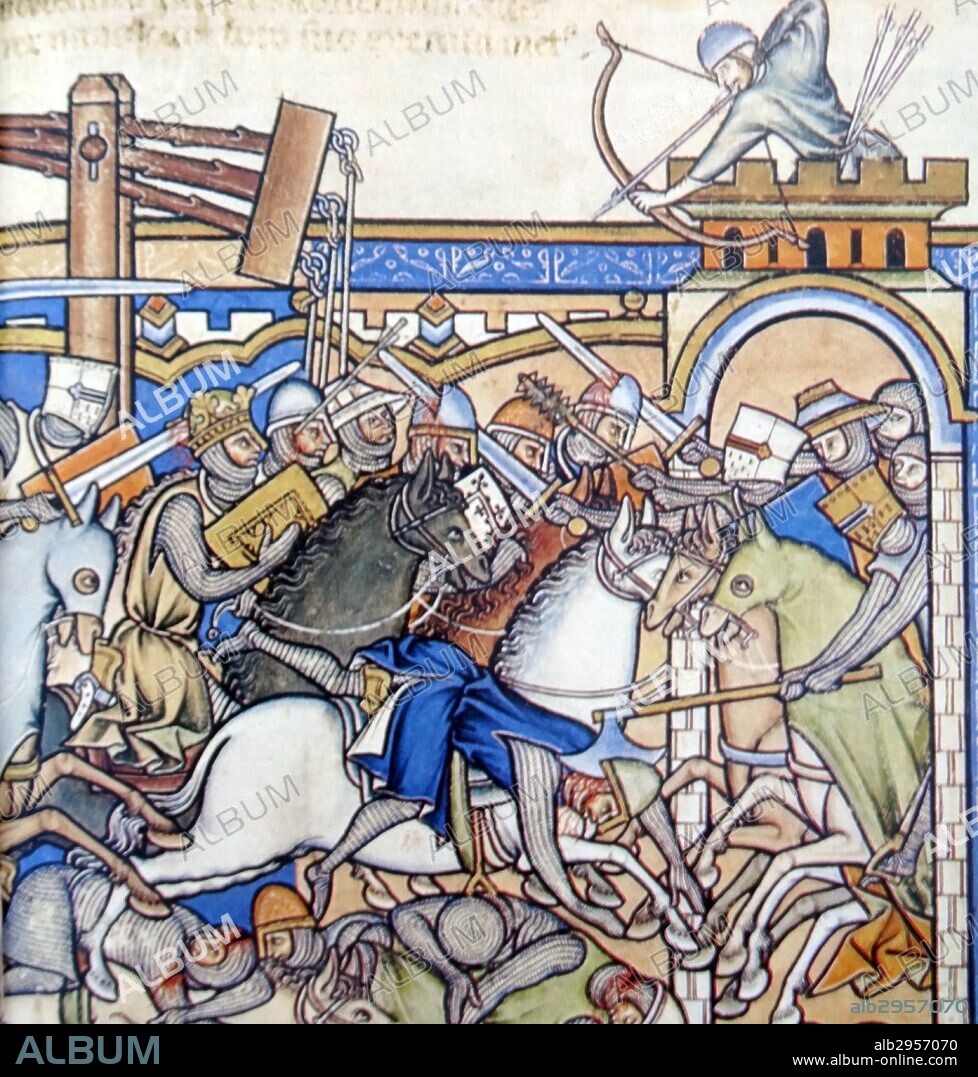The image depicts a vivid and chaotic medieval battlefield, rich in colorful illustration and stained glass-like artistry. Soldiers in armor, some mounted on brown, white, and a prominent black horse, engage in intense combat outside and within the confines of a stone fort. An arched doorway, partially camouflaged, serves as a key point of defense, guarded fiercely by warriors. Atop a tower, an archer aims his bow, with three additional arrows in his belt, ready to rain more attacks upon the intruders below. Around him, the chaos unfolds with men wielding swords, maces, and axes. A trebuchet, etched in brown, stands ready to launch its devastating payload. The scene is marked with graphic detail—blood spurting from wounds, warriors striking mortal blows, and the visceral struggle for control. High above and below the image, a watermark reading "Albem" appears in gray, while a black bar at the bottom includes additional text and a website link, reinforcing the theme of medieval warfare.